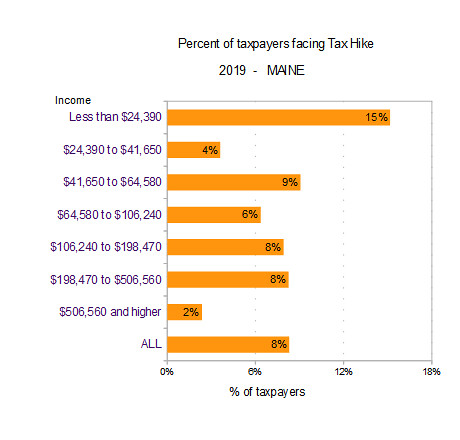The image features a detailed horizontal bar chart centered within it, titled "Percent of Taxpayers Facing Tax Hike, 2019 - Maine." The chart, which is primarily black, white, and orange, resembles those commonly found on government or news websites. Positioned on the x-axis are the percentages: 0%, 6%, 12%, and 18%, while the y-axis lists various income ranges, beginning with "Less than $24,390" and ending with "$506,560 and higher." Each bar is orange, with corresponding percentages displayed within them. Notably, the income range "Less than $24,390" has the highest percentage at 15%, while the "$506,560 and higher" range shows the lowest at 2%. Other income ranges and their respective percentages include: $24,390 to $41,650 at 4%, $41,650 to $64,580 at 9%, $64,580 to $106,240 at 6%, $106,240 to $198,470 at 8%, and $198,470 to $506,560 also at 8%. An overarching category, "All," indicates an 8% tax hike for all taxpayers.